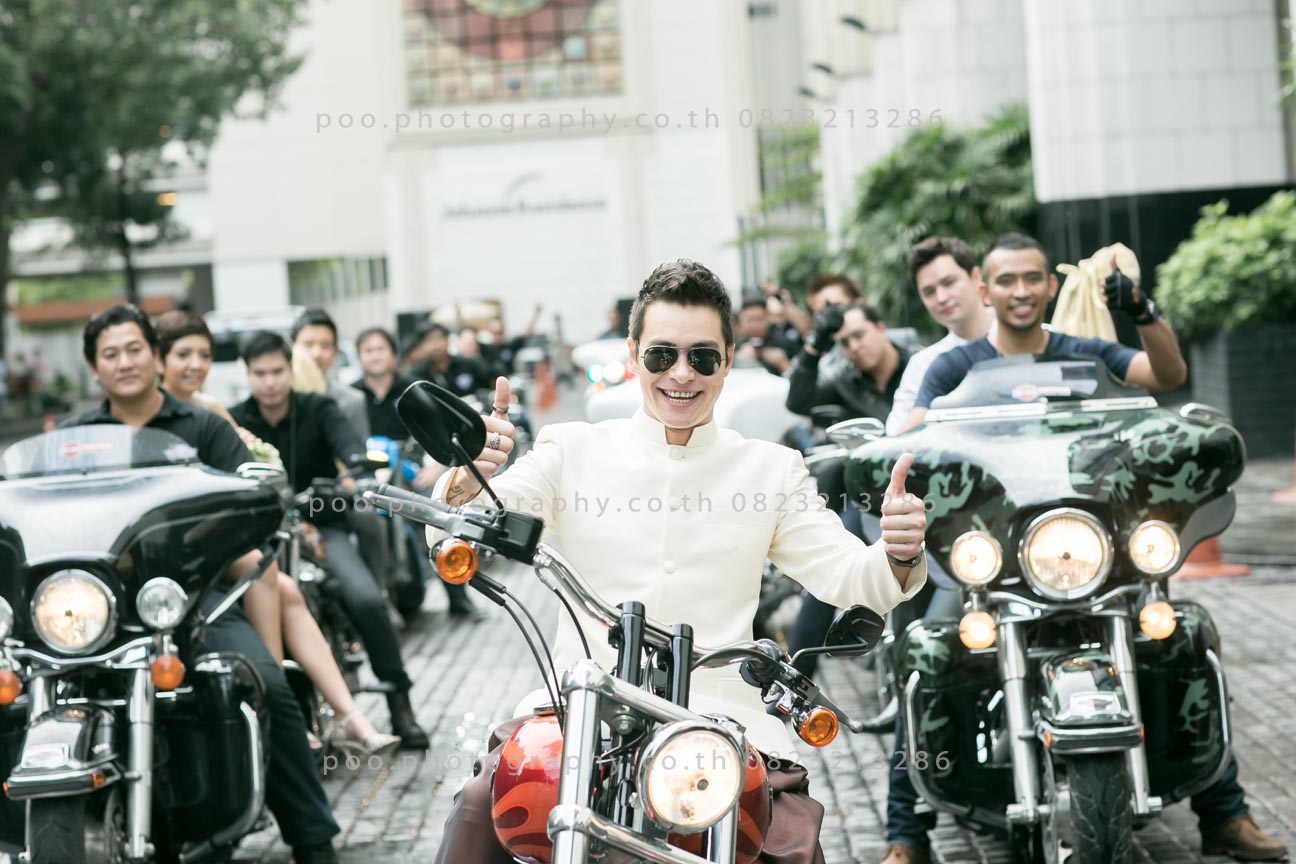This landscape photograph captures a vibrant motorcycle procession, potentially part of a wedding or an advertisement for a photography company. At the forefront, a man dressed in a white shirt and black sunglasses, with dark hair, is the main focal point. He is riding a striking red and orange motorcycle adorned with flames on the gas tank, confidently giving a double thumbs up to the camera. Surrounding him are rows of around ten more riders on motorcycles, which gradually become blurrier as they recede into the background. To the left of the main figure, another man shows a thumbs-up sign, riding a larger green and black camouflage motorcycle, while to his right, a rider on a black motorcycle remains without any gestures. Most individuals in the procession, all appearing to be men or short-haired people, display varying expressions from forward-looking stoicism to enthusiastic smiles. They ride on what seems to be a cobblestone or gray paved road, framed by a white building and blurred greenery, trees, and planters, adding a lush backdrop to the lively scene.